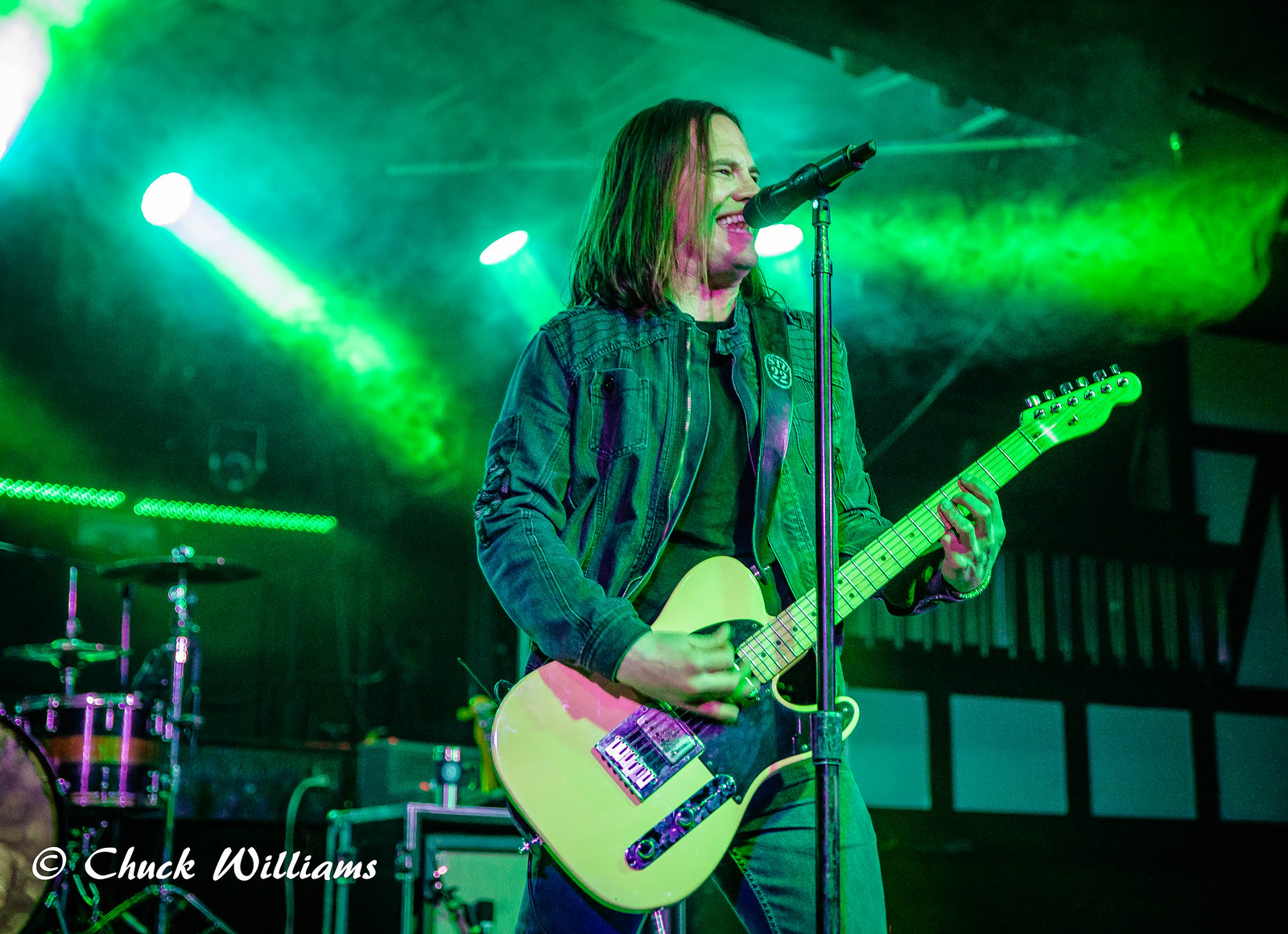This photograph, taken by Chuck Williams and clearly marked with his copyright in the lower left-hand corner, captures a white man in his 30s, likely a musician, performing on stage inside a concert hall. He has long, shoulder-length hair and is dressed in a denim jacket, black t-shirt, and blue jeans. The man stands in front of a microphone—mounted on a stand—smiling and possibly singing as he plays a light wood-colored electric guitar with a dark wood highlight. The stage is bathed in green light, casting a green tint over the scene, and smoke enhances the atmospheric effect. In the background, a partial drum set is visible along with some stereo equipment and spotlights shining through the green smoke.